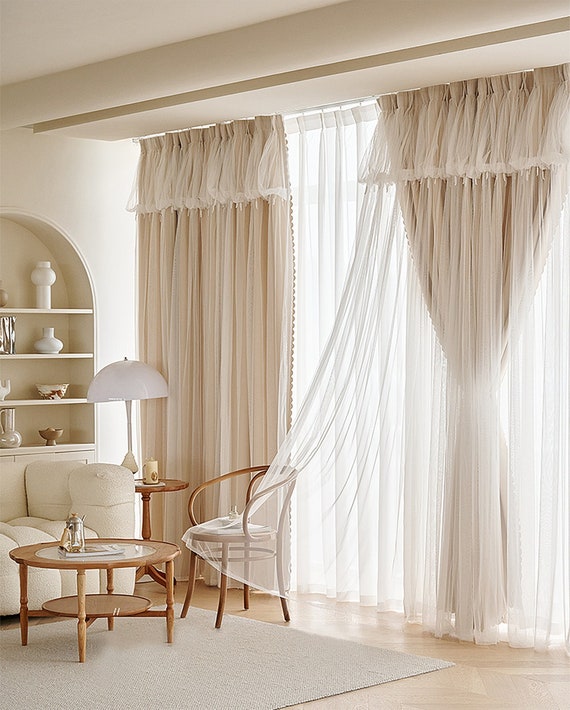The image showcases a minimalist living room bathed in neutral, muted tones. Dominating the right side of the room is a large window adorned with sheer white and beige curtains, through which soft light filters. The room features white and cream walls, with a mix of beige, brown, and white elements throughout, contributing to a cohesive color scheme.

To the right of the window stands a brown wooden chair partially covered by one of the curtains. In front of this chair, a small round wooden table supports a book and a silver Kintsu. Adjacent to the chair is a white sofa, accompanied by a side table with a round white lamp on it. The lamp, featuring a wide, rounded shade, is placed next to a white mug.

Central to the room is a cream-colored rug on top of wooden brown floors. A coffee table, also brown, sits atop the rug, maintaining the room's earthy palette. In the background, a series of four shelves display various vases and bowls in white, beige, and brown hues, all against a cream-colored wall. The design speaks to a harmonious blend of simplicity and elegance, with each element contributing to the overall serene ambiance.